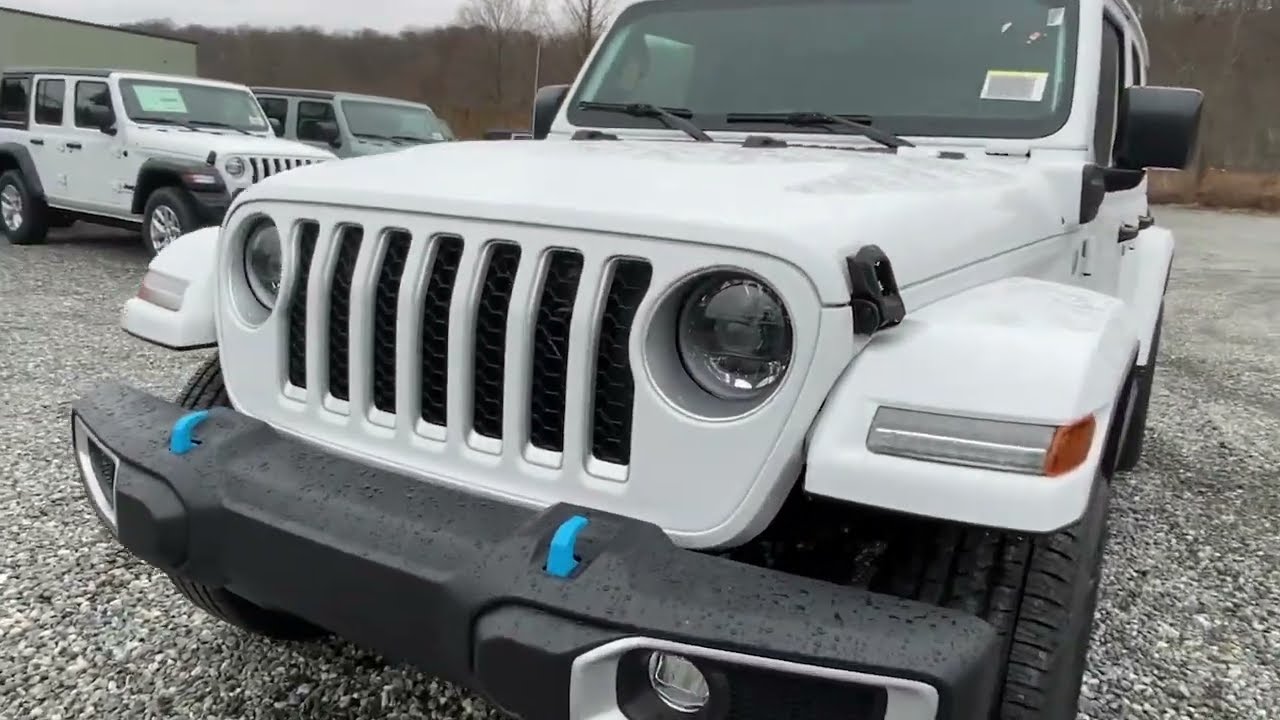In this rectangular image, there is a close-up view of the front of a white vehicle that appears to be an all-terrain truck or possibly a station wagon, parked diagonally to the left. The truck features a black bumper with two distinctive blue hooks. Only the front two black tires are visible. The vehicle sits on a bumpy gravel road covered in multicolored, small gray rocks. The gravel appears damp, suggesting it has recently rained, and there are raindrops visible on the vehicle’s front. The sky is overcast and gray, adding to the gloomy atmosphere. In the background, there are two similar vehicles; one is white and the other is grayish-green. These vehicles are parked on the left behind the primary truck. A row of leafless, brown trees can be seen further back, indicating a forest of dead trees. On the upper left, the faint sky is visible, and to the right, there is a nondescript beige building partially obscured by the vehicles. The absence of people and the overall setting evoke a sense of desolation and abandonment.